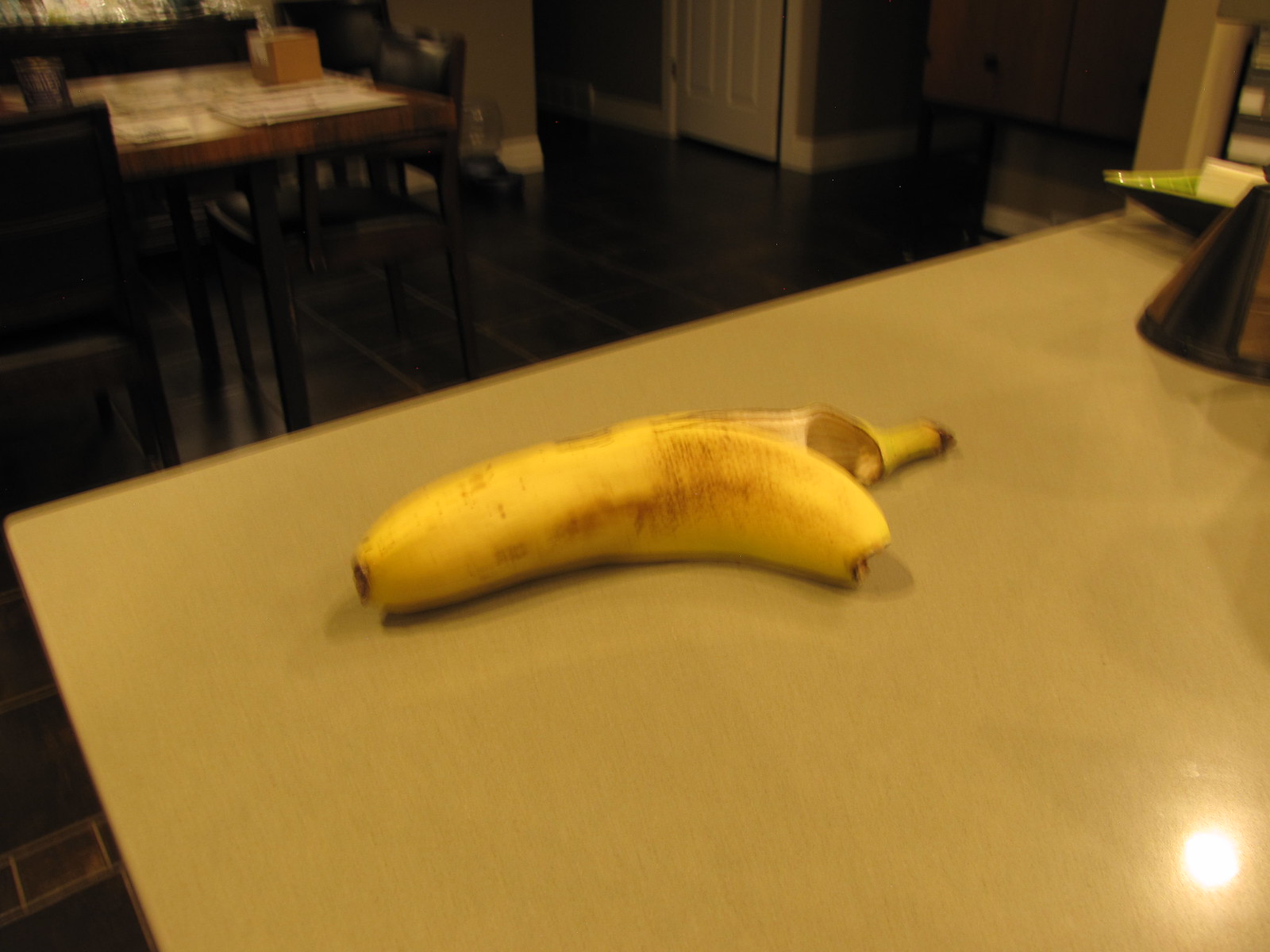A blurry photograph captures a half-peeled banana resting on a countertop, illuminated by somewhat dark and greenish-yellow lighting. The countertop itself appears to be a mix of greenish-gray and yellow hues, with a reflective spot of light noticeable in the bottom right corner. The banana peel, occupying the center of the image, is bright yellow with brown speckles, split into two halfway down. On the countertop, to the right of the banana, there is a cone-like object and a square dish containing something white. In the background, the image softly transitions into a dining area, featuring a dining table with black chairs adorned with placemats. The floor is tiled in black, and a cat feeder is visible near the hallway, which leads to a white door and continues further to another indistinct doorway. The overall scene is blurred and tinged with a greenish-yellow light, making the details appear hazy.